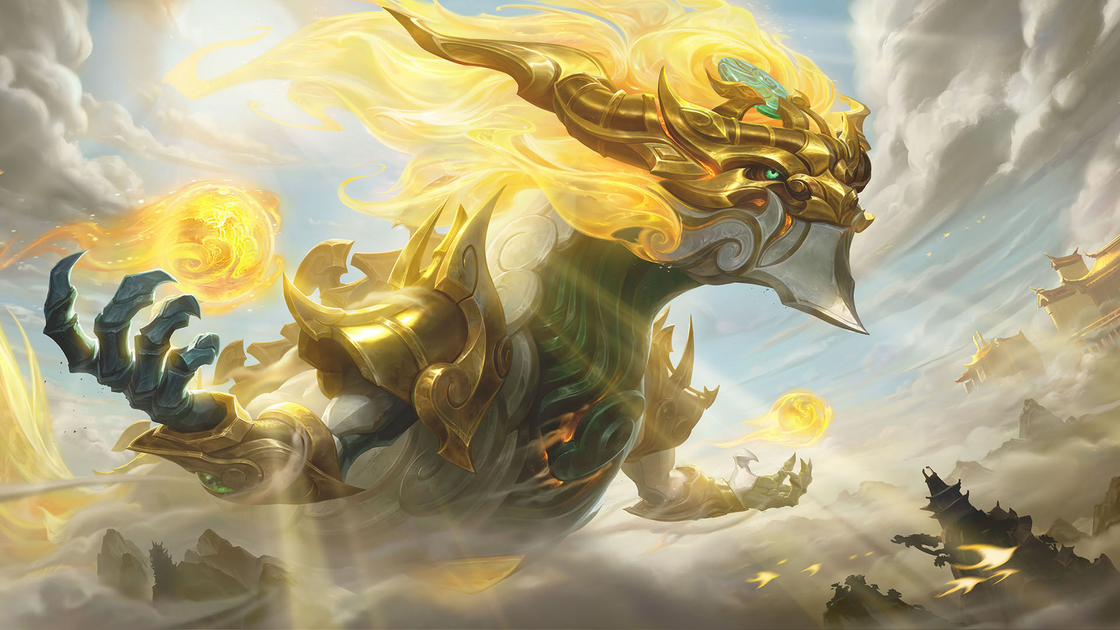The image depicts a computer-generated, animated scene featuring a large, dragon-like monster with sharp, pointed features and vibrant details. The background showcases dynamic, wispy clouds in various shades of gray, suggesting strong winds. The monster, centrally positioned, has yellow, fire-like hair and golden horns, emphasizing its fierce appearance. Its eyes gleam green, matching a jade turquoise apparatus on its head. The creature has elongated, blue claws, and in one of its claw-like hands, it holds a fiery orb. The scene also includes hints of rocks, mountains, trees, and what appears to be an ancient dragon lair in the bottom right corner. The monster's white, protruding chin, and armor-like gold top add to its intimidating presence, with the entire image rendered in muted tones of yellow, gray, and beige, intensifying the dramatic and otherworldly atmosphere.